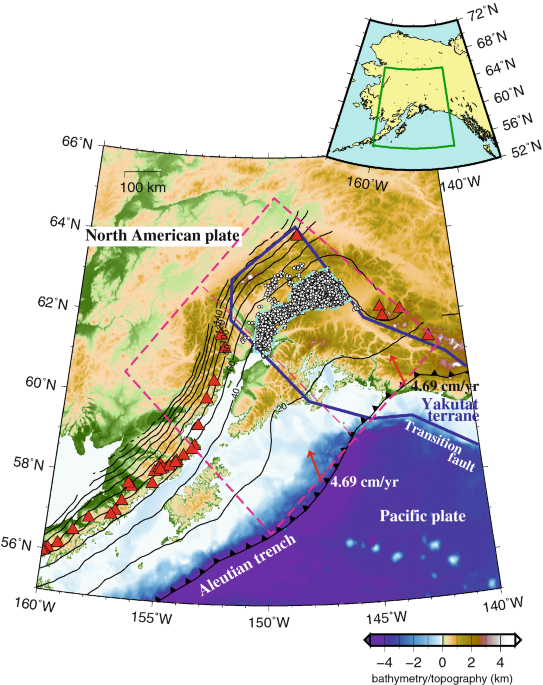The image depicts a detailed geographical and topographical map of Alaska, with specific focus on the tectonic plates and fault lines within the region. The map is predominantly green and brown, with additional markings in pink and red to highlight specific features. At the upper right corner, there's a smaller overview map of Alaska, with a green box indicating the zoomed-in area featured below. The main map highlights the North American Plate and includes various labels such as the Aleutian Trench, Pacific Plate, Transition Fault, and Yakutat Terrane. It shows detailed latitude lines ranging from 56°N to 66°N and longitude lines from 140°W to 160°W. The map details bathymetry and topography measurements in kilometers, indicated by a color scale from dark blue to white. Specific features like red triangles along the Aleutian Islands suggest tectonic activity, with annotations such as "4.69 cm/year" providing additional geological context.